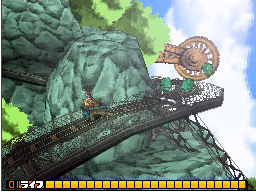The image is a colorful screenshot from a computer game, featuring a detailed scene with several distinct elements. At the bottom of the screen, there's a section with yellow squares rimmed in black, displaying the number "517" in white, accompanied by a hint of orange. The central focus is a character walking upwards along a long, black pathway or bridge. The bridge leads to a circular, gear-like section colored in red. Large stones are scattered around the character as he progresses, and in the distance, trees are visible against a backdrop of a blue sky filled with white clouds. Additionally, some kind of fencing extends from the bridge, though its exact nature is unclear.